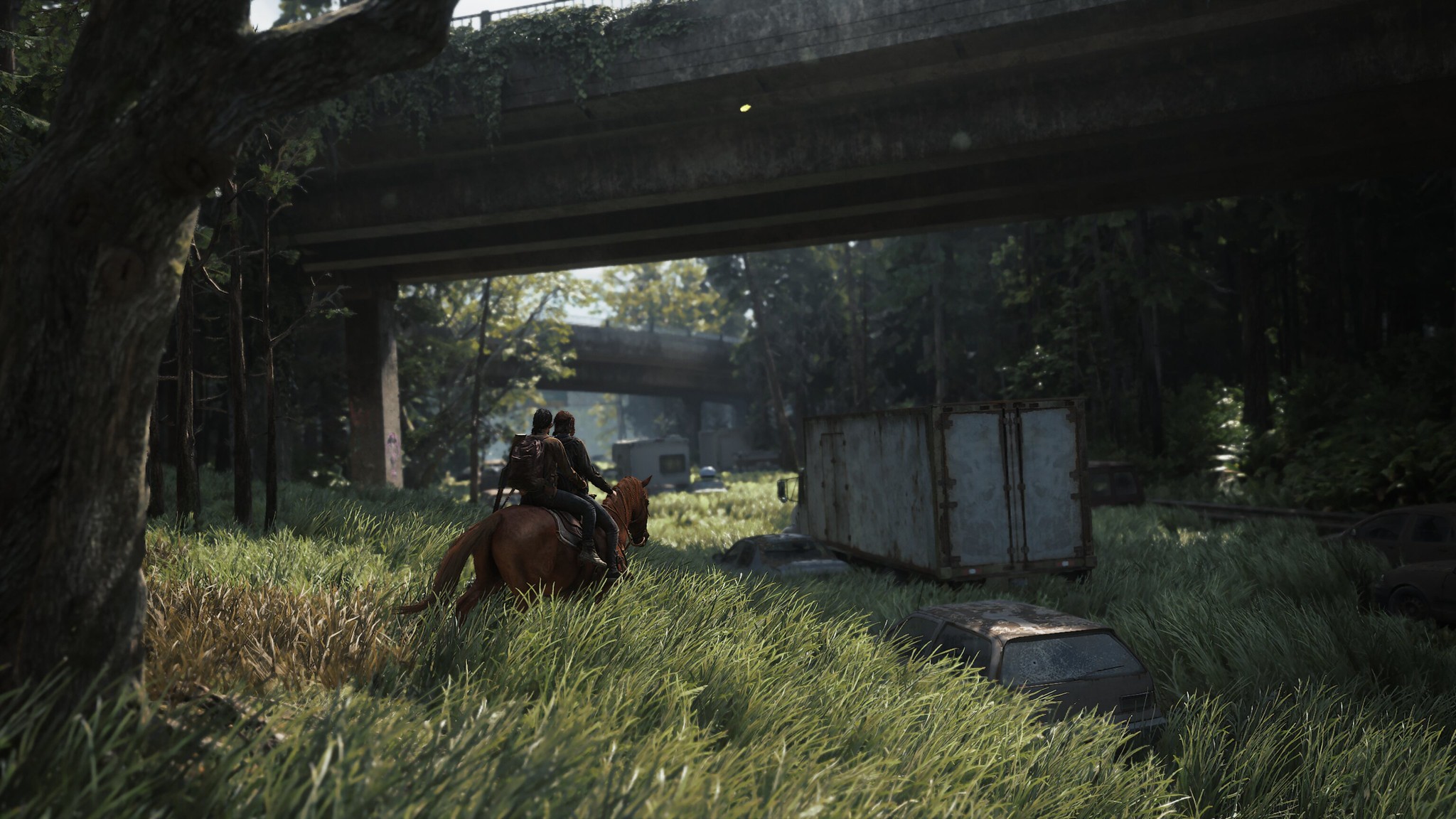In the dimly lit outdoor scene, two men, both clad in long pants and dark shirts, are seen riding a brown horse away from the camera, making their faces indiscernible. They traverse through an expanse of tall, green grass that reaches up to the horse's belly. Above them, an old, weathered bridge extends overhead. To the left, a sturdy tree trunk rises prominently from the ground. In the background, another decrepit bridge is faintly visible, evoking a sense of abandonment. Nestled in the bottom right corner of the image, an old, abandoned car lies partially obscured in a gully, adjacent to a gray, metallic box or item of similar size. The overall atmosphere is one of quiet desolation amidst the natural setting.